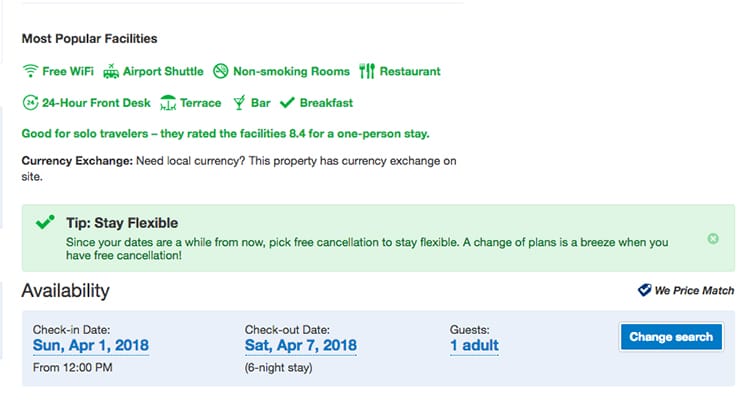The image features a white panel across the top with black lettering. On the left-hand side, it lists the most popular facilities available, illustrated with green icons and symbols, including free Wi-Fi, Airbus shuttle, non-smoking rooms, restaurant, 24-hour front desk, terrace, bar, and breakfast. Below these amenities, there's text in green highlighting that the property is "Good for solo travelers" with a rating of 8.4 for a one-person stay.

Beneath this, in bolded black text of the same size, the property indicates that they offer currency exchange services with an accompanying statement: "If you need local currency, this property has currency exchange on site."

Centered within the image is a green panel containing a tip, marked by a tick symbol: "Stay flexible. Since your dates are a while from now, pick free cancellation to stay flexible. A change of plans is a breeze when you have free cancellation."

Towards the bottom left, the word "Availability" is prominently displayed in a large black heading. Directly beneath it, a blue panel spans across the image with clickable links for "Check-in date," "Check-out date," and "Guests." To the right of these links is a blue "Change search" button, allowing users to modify their search criteria.